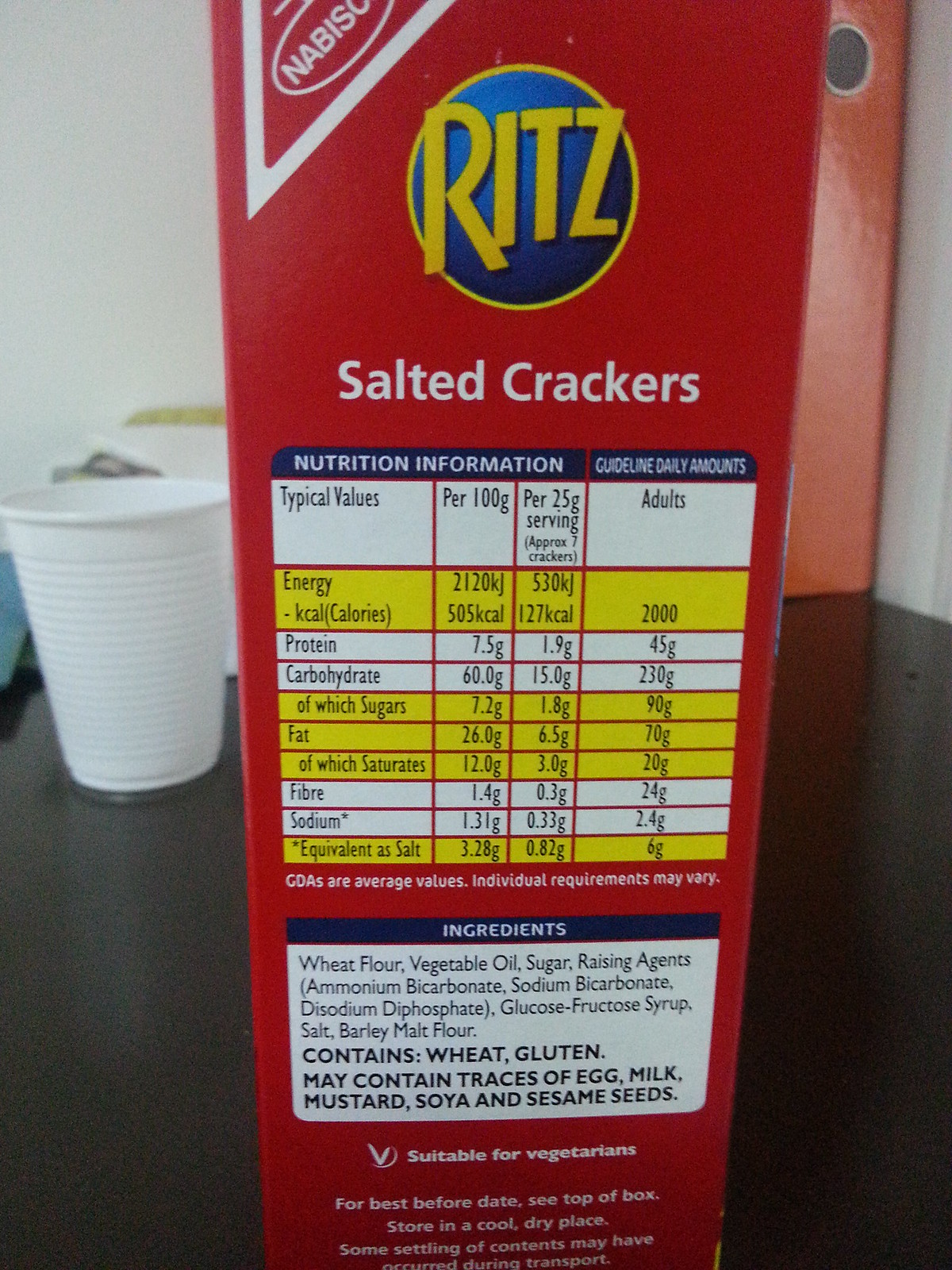A close-up photograph showcases the side of a vibrant Ritz cracker box, positioned on a black Formica tabletop. The iconic packaging features a striking royal blue circle with a gold border, prominently displaying the gold letters "Ritz." Beneath this, the words "salted crackers" appear in white letters. Lower on the box, the detailed nutrition information panel is visible, featuring alternating lines of white and yellow values, separated by thin red lines. Below the panel, within a white rectangle and topped with a blue banner, the word "ingredients" appears in white letters, followed by the ingredient list in blue.

Adjacent to the box, a white plastic drinking cup sits on the table, with a small pool of liquid forming underneath it. In the background, on the opposite side of the box and set against the wall, there's an object in a glossy red color, adding a splash of brightness to the scene.